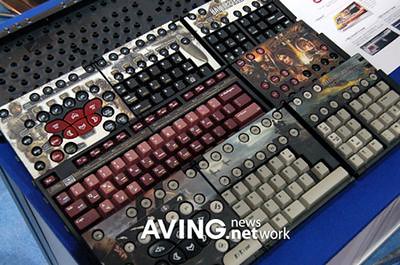The image presents a detailed workspace scene showcasing an assortment of keyboards, seemingly arranged for cleaning or artistic display. At the center, there's a keyboard stripped of all its keys, revealing a black surface with a brushed steel or aluminum backing. This keyboard is positioned slightly behind another one that features a mix of red and black keys, with some form of military-themed overlay displaying personnel and possibly the words "battle foot."

To the left, there's another keyboard sporting pink and maroon keys along the left side and top row, covered by a skin depicting an arcane-looking woman with long brown hair engaged in some magical activity. Scattered about are black and red buttons. Another keyboard to the far left has unconventional round keys alongside typical ones, possibly resembling an art piece with remote-control-like special keys.

The lower part of the image has a caption that reads "aving.newsnetwork," linking to "Aving.net," suggesting some artistic installation or custom-painted keyboards. A keyboard in the bottom left area features white keycaps, a white number pad, and directional arrow keys in black. On the surface, there are various documents stacked in the upper right corner, and the base is a blue surface with white accents.